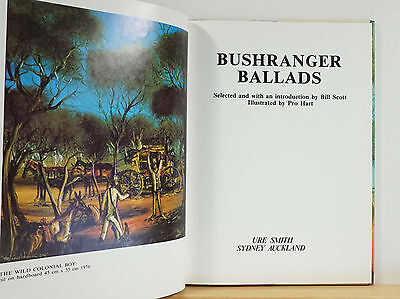This photograph captures an open book resting on a brown wooden floor and leaning against a plain white wall. The left-hand page features a detailed illustration, depicting a bright blue sky with distinct Australian trees and a horse-drawn carriage. In the foreground, a dramatic scene unfolds: a man with his hands raised is being confronted by another man emerging from the forest with a donkey and pointing a gun. Above this vivid depiction, in all caps, the title "The Wild Colonial Boy" is prominently displayed. The right-hand page, in stark contrast, comprises mostly text. At the top, in bold capital letters, it announces, "BUSH RANGER BALLADS," followed by the inscription, "Selected and with an Introduction by Bill Scott, Illustrated by Pro Hart." The bottom of the page bears the names "URI SMITH" and "SYDNEY AUCKLAND" in black lettering. Overall, this image suggests a book rich in historical ballads from Australia, with the text on the right side indicating a curated and illustrated collection of bushranger stories.